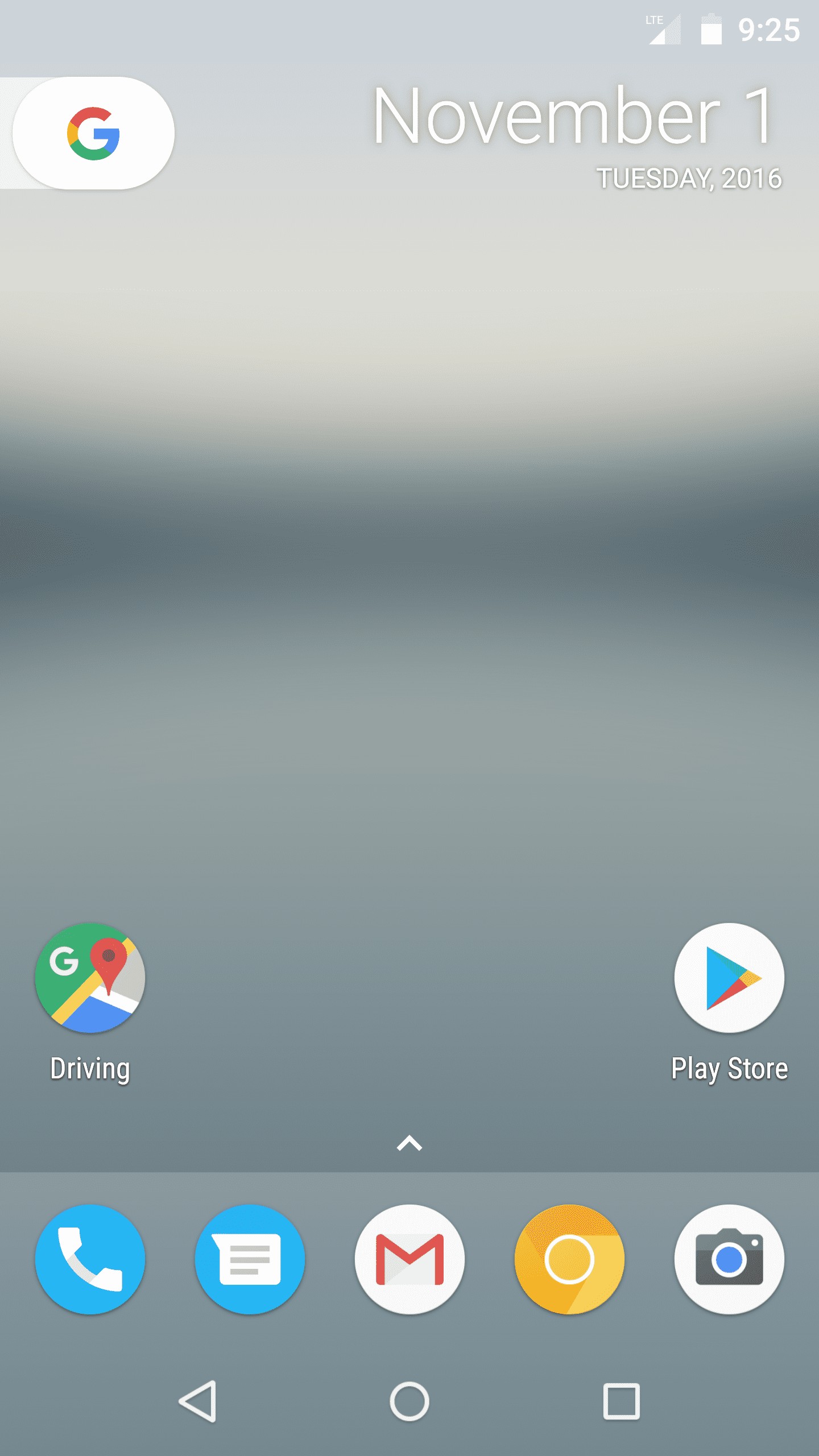The image is a screenshot of a smartphone's home screen. At the top left corner, there is the Google logo (G). On the right side, the date is displayed as "November 1st, Tuesday 2016". Above the date, the time is shown as "9:25". Next to the time, there is a nearly full battery icon, alongside the data connectivity bars.

At the bottom of the screen, on the left side, there is a widget labeled "Driving" with its corresponding app icon. On the bottom right, the Play Store app icon is visible. The very bottom row features a row of app icons: Phone, Messaging, Gmail, Chrome, and Camera.